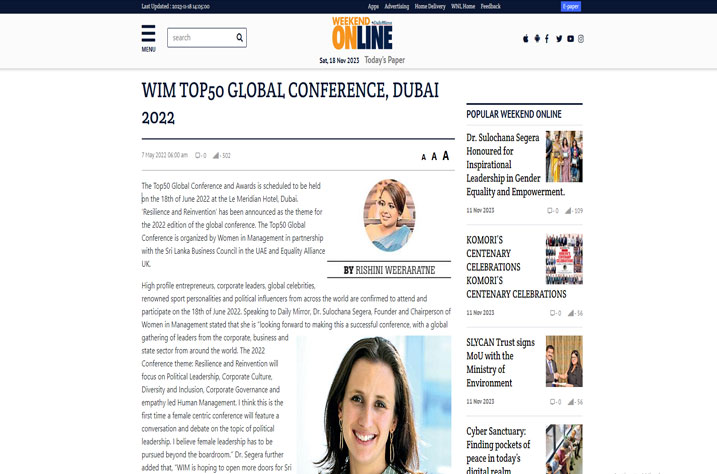The image portrays a webpage, presumably a blog or website, with various elements organized in a clean, user-friendly layout. At the very top, a thin black bar spans the width of the page, featuring a series of tabs on the left side indicating "Last Updated" along with a timestamp and date information. The central portion of this top bar lists some app-related links, and on the far right, there are additional small, somewhat difficult-to-read tabs.

Beneath this black bar, a banner prominently displays the site name "Weekend Online," with "weekend" in orange, "on" in orange, and "line" in blue. Below this banner, the current date is displayed: "Sunday 15th of November 2023." Adjacent to the date, social media icons allow for easy sharing and connectivity.

On the left, a menu button facilitates navigation, accompanied by a search bar for quick content discovery. The main article featured on the page is titled "W.I.M. Top 50 Global Conference Dubai 2022," authored by Rashini Riratini.

To the right of the main article, a side panel lists "Popular Weekend Online Articles," offering readers quick access to other trending content on the site. The elements are carefully structured to provide a seamless browsing experience while keeping important information readily accessible.